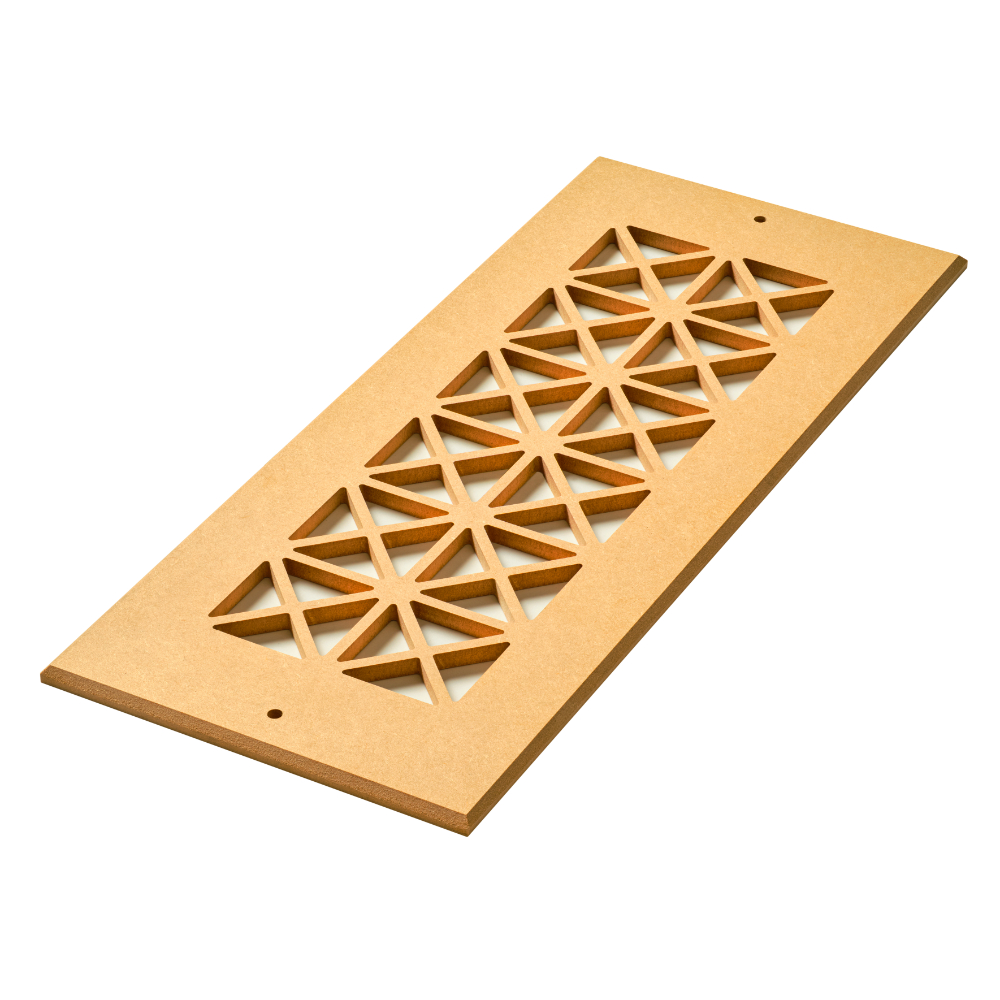The image depicts a light brown wooden panel with a decorative design, angled from the bottom left to the top right of the picture. The central focus of the panel features a 2 by 6 grid of cut-out X patterns, each intricately crafted to appear three-dimensional with careful shading and dark outlines. These outlines create a sense of depth, enhancing the textured look of the wood. The panel, which resembles the size of a light switch cover, includes a screw hole at each end—one at the top and one at the bottom—suggesting that it is meant to be mounted. The background of the image is plain white, highlighting the detailed craftsmanship of the wooden panel. Despite its detailed design, the panel appears to lack a specific functional purpose and might simply serve as a decorative piece.